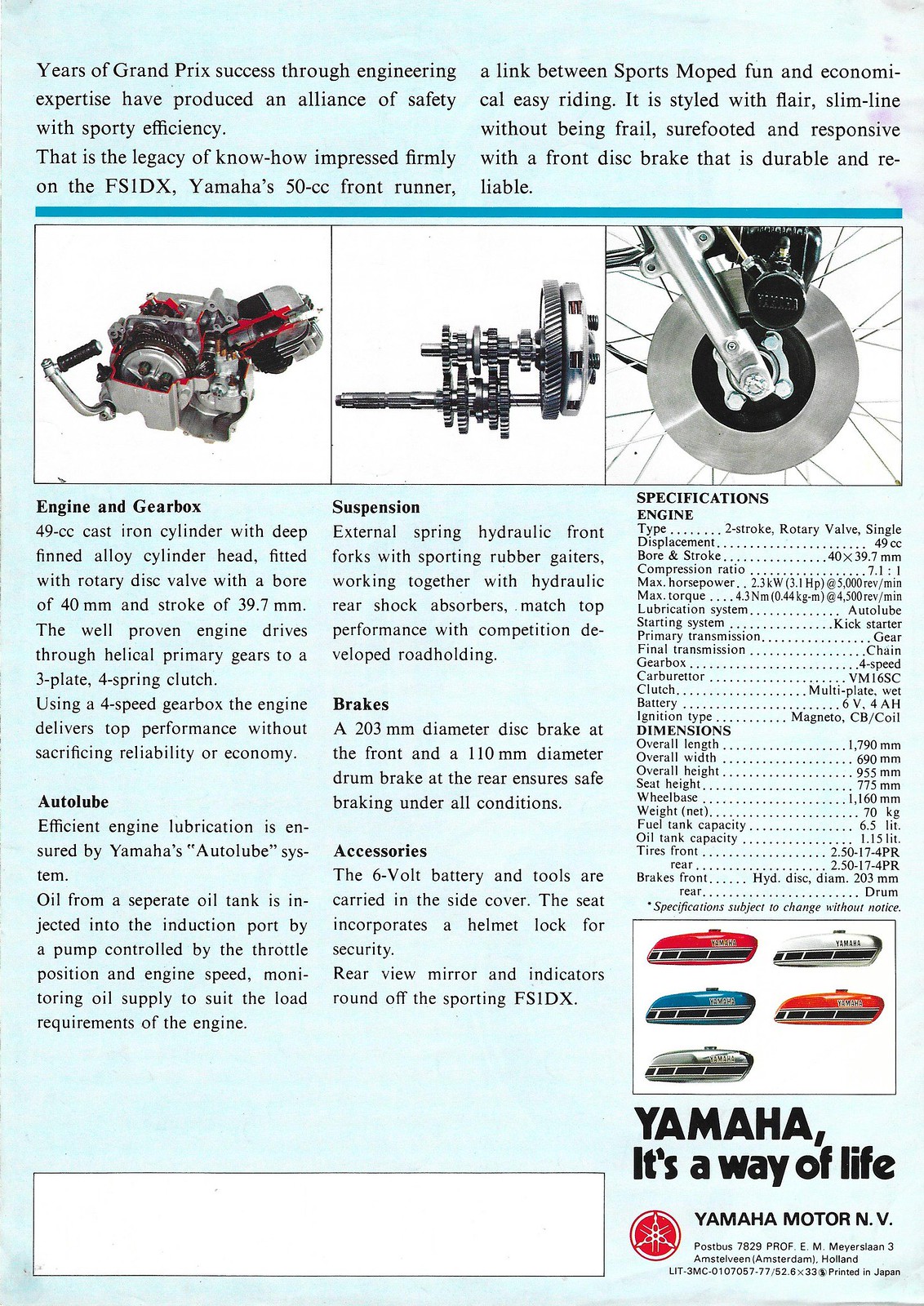This advertisement for Yamaha prominently features a detailed and technical display of the Yamaha FS-1DX moped, emphasizing the company's legacy of engineering excellence and Grand Prix success. The page, captured in a portrait orientation with a light blue background, is divided into several sections for clarity.

At the top, three side-by-side images with a white background depict various motorcycle components, including a motor, a wheel, and gears. These images are accompanied by a blue rule across their tops and are overlaid with two columns of text in black. The text celebrates Yamaha's engineering expertise, highlighting the blend of safety, sporty efficiency, and years of Grand Prix success that defines the FS-1DX Yamaha's 50cc front-runner. This moped is noted for its stylish yet robust design, featuring a durable and responsive front disc brake.

Below these images, three columns of black text provide in-depth descriptions of the moped's features:

1. **Engine and Gearbox**: This section details the moped's 49cc, cast iron cylinder engine with deep finned alloy cylinder head, fitted with a rotary disc valve. The engine is driven through helical primary gears to a three-plate, four-spring clutch, ensuring top performance without compromising reliability and economy.

2. **Suspension and Brakes**: Here, the ad describes the external spring hydraulic front forks with rubber gaiters, paired with hydraulic rear shock absorbers for superior road holding. Safe braking is ensured by a 203mm diameter disc brake at the front and a 110mm diameter drum brake at the rear.

3. **Specifications**: This column, akin to a technical table, lists detailed specifications, such as the two-stroke rotary valve engine, 2.3 kW (3.1 horsepower) at 5000 RPM, auto lube lubrication system, 4-speed gearbox, and dimensions including an overall length of 1790mm, width of 690mm, and weight of 70kg. Fuel and oil tank capacities are 6.5 liters and 1.15 liters, respectively.

In the bottom right corner, a graphic of what appears to be motor parts is visually linked to the technical details provided. Adjacent to this graphic, text proclaims "Yamaha, It's a Way of Life," accompanied by the Yamaha Motor NV logo and additional location and contact details. A red circle resembling a tire wheel is positioned to the left of this information, and a blank white horizontal box is evident at the bottom left, contributing to the clean graphic design of the page. The publication note, "Specifications subject to change without notice," is subtly placed to remind readers of possible updates.